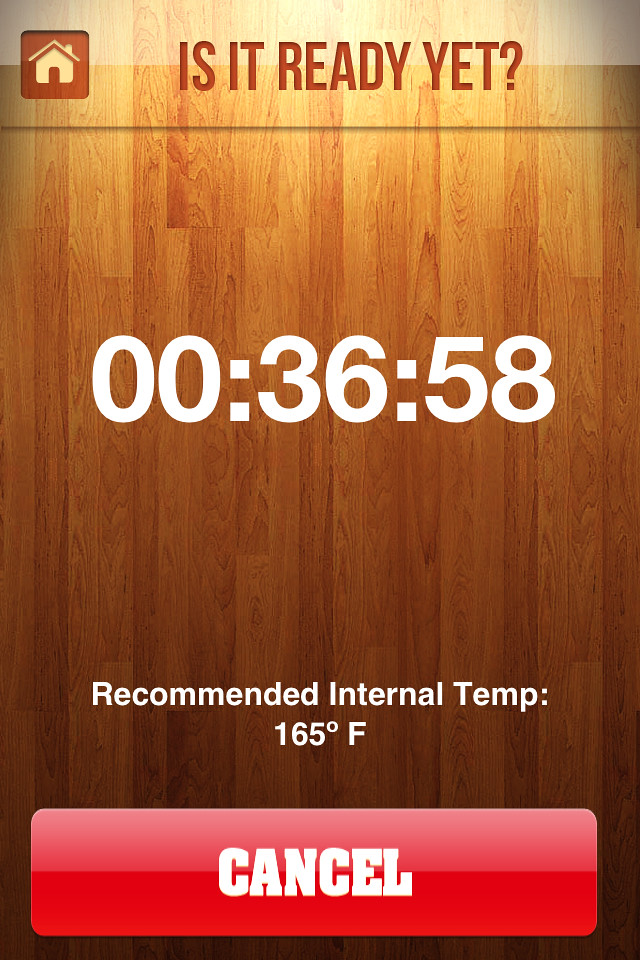The image resembles an advertisement, possibly for a mobile application, featuring a user interface set against a wood-grain background. The background transitions from a lighter wood at the top to a darker stain at the bottom. At the top, there's a subtle white translucent border. In the upper left corner, a home-shaped button, resembling a carved icon, is embedded into the wood. Carved lettering at the top reads "Is it ready yet?" followed by a timer displaying "00:36:58". At the bottom, white text indicates "Recommended internal temp: 165°F." A prominent red button with white lettering reading "CANCEL" is located at the bottom of the image.